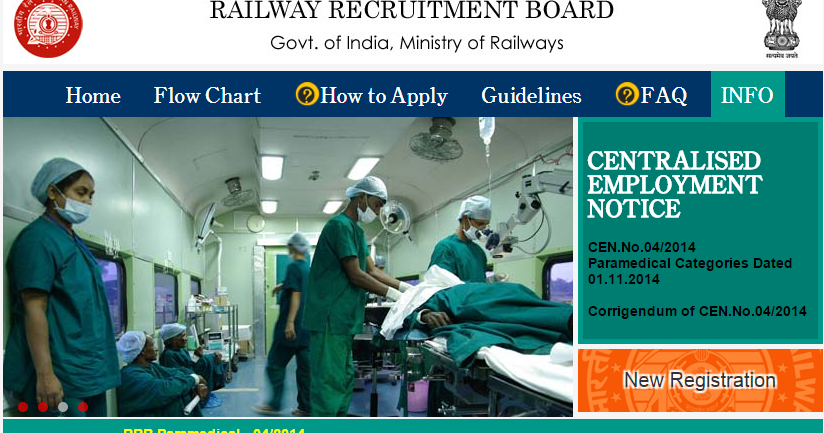Here is the refined and descriptive caption for the image:

---

The webpage prominently displays the title "Railway Recruitment Board" in large, bold, black capital letters at the top center. To the left of the title is a red crest with an intricate central design set against a white background. On the opposite side, to the right, there is an emblem resembling a vase, characterized by a rounded base that narrows as it extends upward. This emblem is labeled with the text "Government of India, Ministry of Railways."

Below the central title, there is a photograph depicting a scene from a medical facility. The image captures multiple members of medical staff wearing masks. Some staff members are seated, while a young woman leans against the wall, and another person is visible walking in the background. The focal point of the photograph is two doctors attending to a patient lying on a gurney.

Additionally, the page features textual details about a "Centralized Employment Notice" with the CEN number "4-2014," dated 1-11-2014. A related amendment or corrigendum, referencing the same CEN number, is noted with the date 4-20-2014. An orange box labeled "New Registration" appears on the right side of the page. The view of the webpage cuts off at the bottom, truncating any further content.

---